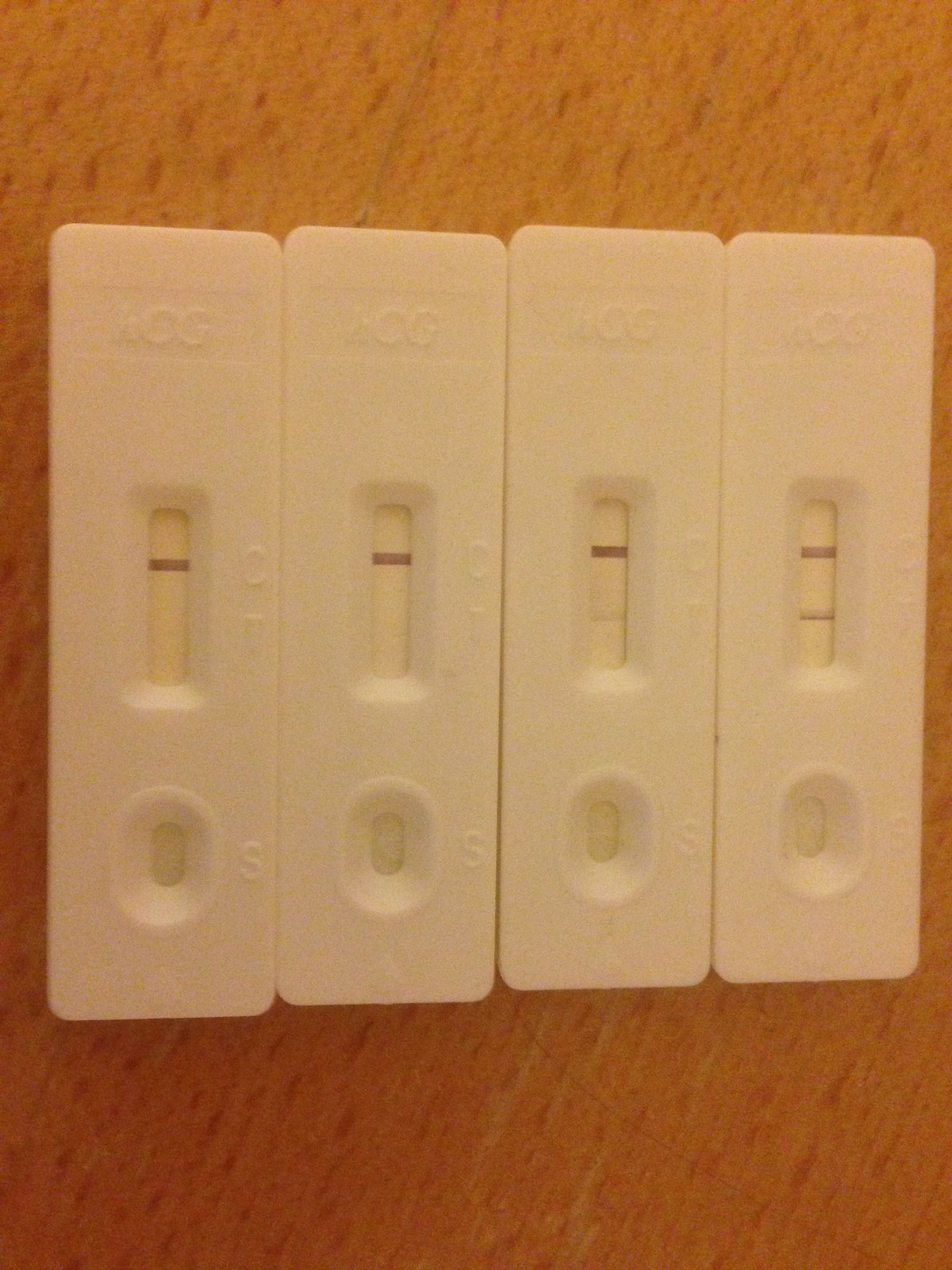This image features a close-up view of four HCG tests arranged in a row, spanning from left to right across a brown table adorned with darker brown flecks in its grain. Each HCG test is an elongated white plastic device, clearly marked with "HCG" at the top. Below the marking, the tests have a small rectangular viewing window with visible lines and partially obscured stamped letters beside it. Further down, there is a circular spot designed for applying the fluid sample.

The first two tests on the left display only the control line, indicating a negative result. The third test shows a control line as well as a faint line beneath the test indicator (T), suggesting a possible positive result. The fourth test on the far right features both a prominent control line and a nearly equally dark test line, confirming a positive outcome.